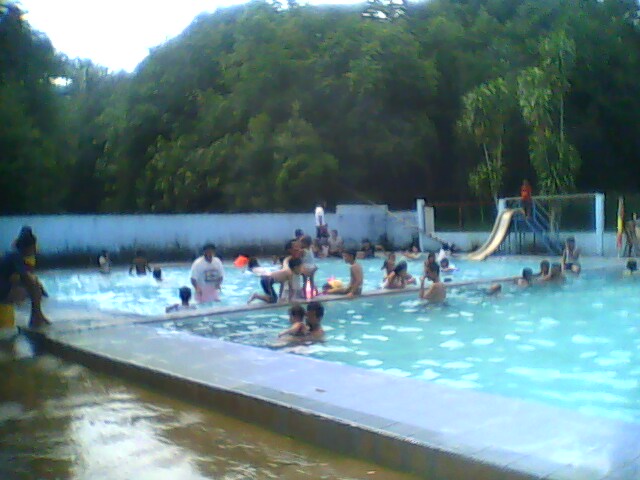The photo captures a bustling outdoor public pool area. Central to the image is a large rectangular in-ground swimming pool, characterized by its light bluish, chlorine-filled water. The pool is sectioned into a deep end and shallow end by a line running horizontally across the water. Adding to the busy scene, numerous people, both adults and children, are seen swimming and playing in the pool, while some kids are crawling and walking on a narrow, cement divider that runs across the water.

To the far right of the pool, a yellow slide with blue steps stands prominently, surrounded by a crowd, including a person at the top preparing to descend. This slide adds a vibrant splash of color amidst the pool's blue and concrete tones. Beyond the pool, tall grass surrounds a white wooden fence, which marks the boundary before a heavily wooded area filled with tall green trees. The sky above is bright, though details of the sun are absent.

Details of the pool area continue with a narrow concrete walkway that stretches from the bottom right corner to the upper left of the photo, with visible signs of wetness from frequent use, indicating a lively, busy day at the pool. The overall image, although slightly blurry, likely due to a wet camera lens, vividly conveys the lively atmosphere of a public pool nestled just at the edge of a forested area.